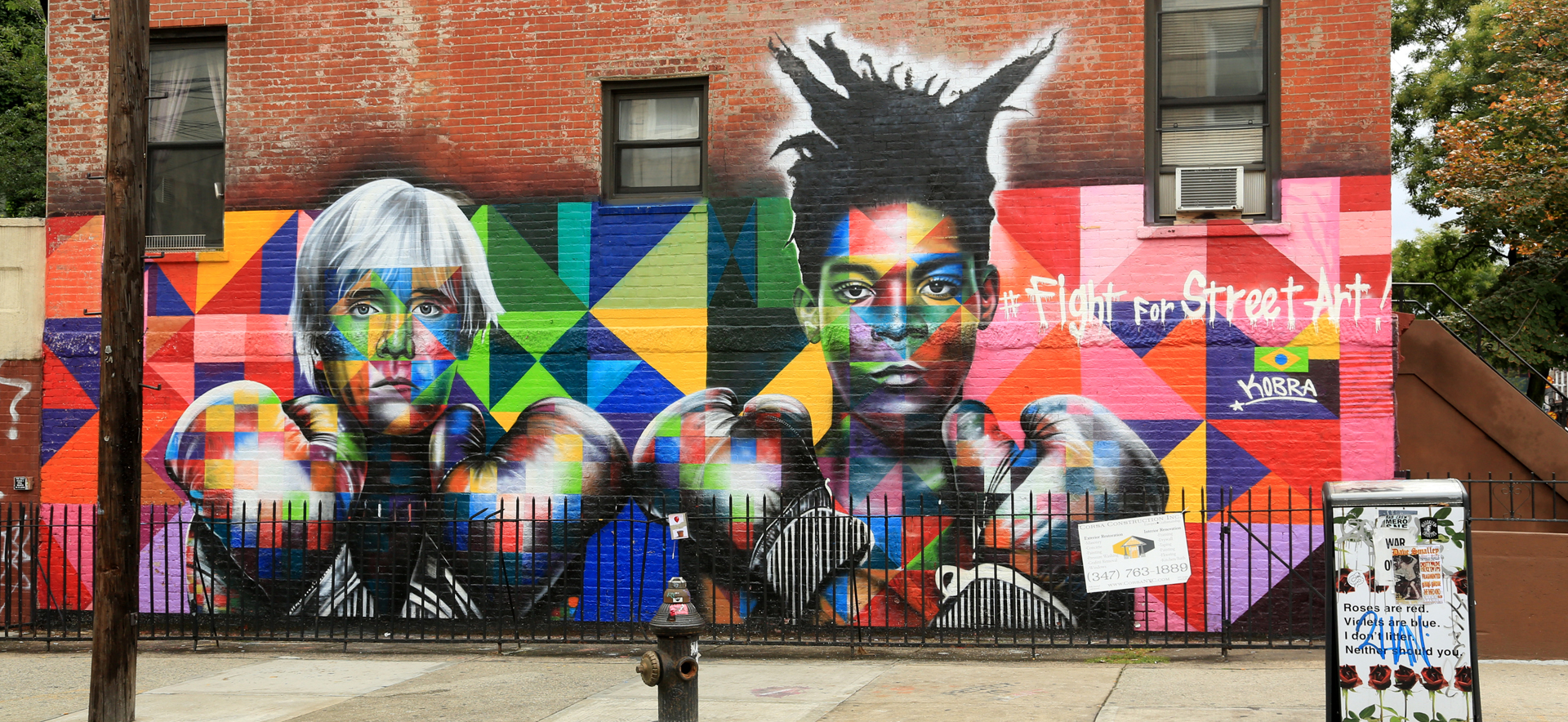The image captures a vibrant graffiti mural on the side of a red brick building in an urban setting. The somewhat faded brickwork, showing patches of tan, contrasts against the mural's lively colors. The mural features two men in black and white, each wearing boxing gloves and crossing their arms over their chest. The man on the left has blonde hair, while the man on the right, who appears African American with dark, spiky or somewhat dreaded hair, has a wide nose and flared nostrils. Both men are looking forward with serious expressions. Surrounding them is a geometric backdrop filled with multicolored triangles and squares in hues of yellows, greens, blues, reds, pinks, and purples. Prominent text near the man on the right declares, "Fight for Street Art," accompanied by a Brazilian flag and the artist's tag, "KOBRA," spelled with a K. In front of the building, a sidewalk houses a black-painted fire hydrant, a display board, a telephone pole, and a black metal fence. On the right side of the frame, stone steps lead up to the building framed by trees with green and reddish leaves. The image, taken in landscape format, reveals the mural as a striking statement on the vibrant, yet gritty, city street.